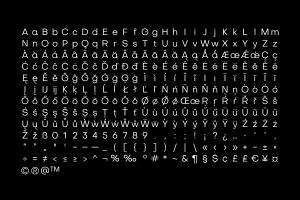The image features a black background with rows of white characters. The first two rows exhibit the English alphabet in both uppercase and lowercase formats: A, a, B, b, C, c, D, d, and so forth, until Z. Following these are rows dedicated to accented letters, starting with different variations of 'A' using diacritical marks from various languages, some stripes composed of solid and dashed lines. Subsequent rows follow the pattern with 'C', 'E', 'U', 'K', 'L', 'N', 'O', 'S', 'T', 'U', 'W', 'Y', and 'Z', each adorned with diverse accents or special characters from different languages. Towards the lower section of the image, the numbers from 0 to 9 are displayed in numerical order. Additionally, there are symbols such as the question mark, its inverted counterpart often used in Spanish, various types of brackets, the equal sign, not equal sign, less than, greater than, and other comparison operators. The image also includes the at symbol (@), copyright symbol (©), and registered trademark symbol (®).